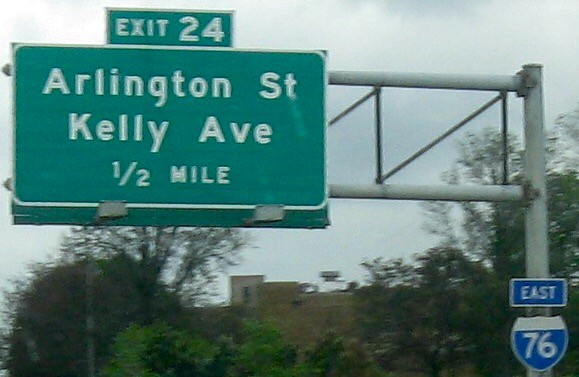This photograph captures a green rectangular highway sign, mounted prominently on a large metal beam structure. Above the main sign is a smaller rectangular sign indicating "Exit 24." The writing on these signs is painted white, with reflective dots embedded in the letters, enhancing visibility at night. The exit leads to Arlington Street and Kelly Avenue, accessible in half a mile. Suspended from the same structure are additional signs: a small rectangular blue sign with "East" in white letters, and below it, an Interstate 76 shield-shaped sign. The background reveals a cloudy sky, a large brick building, and several trees, lending a sense of place to the scene.